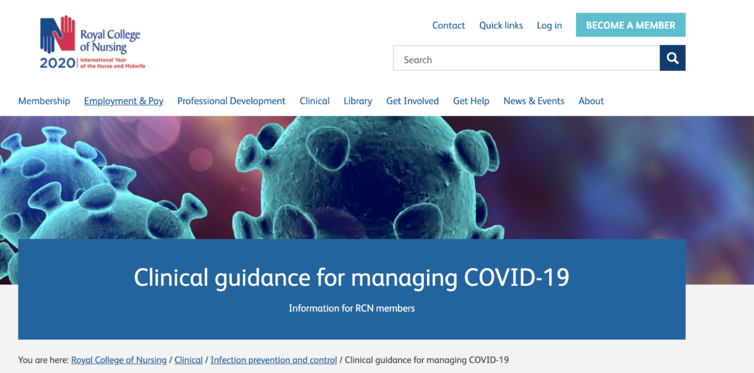Detailed Caption:
A screenshot of the Royal College of Nursing (RCN) website showcasing its resources for COVID-19 management. At the top, the navigation menu includes options such as Membership, Employment and Pay, Professional Development, Clinical, Library, and Get Involved, along with a search bar, contact information, quick links, a login button, and a 'Become a Member' option. Scrolling down, a prominent image of a computer-generated coronavirus, characterized by its distinct spherical body and spike proteins, captures the viewer's attention. The main headline reads 'Clinical Guidance for Managing COVID-19: Information for RCN Members.' Below this, breadcrumb navigation indicates the user’s current path: 'Royal College of Nursing / Clinical / Infection Prevention and Control / Clinical Guidance for Managing COVID.' The webpage predominantly features a white background with gray and blue accents, reinforcing a clean and professional aesthetic. This resource serves as an essential guide for nurses, likely in the UK, given the typical association of a Royal College with British institutions.